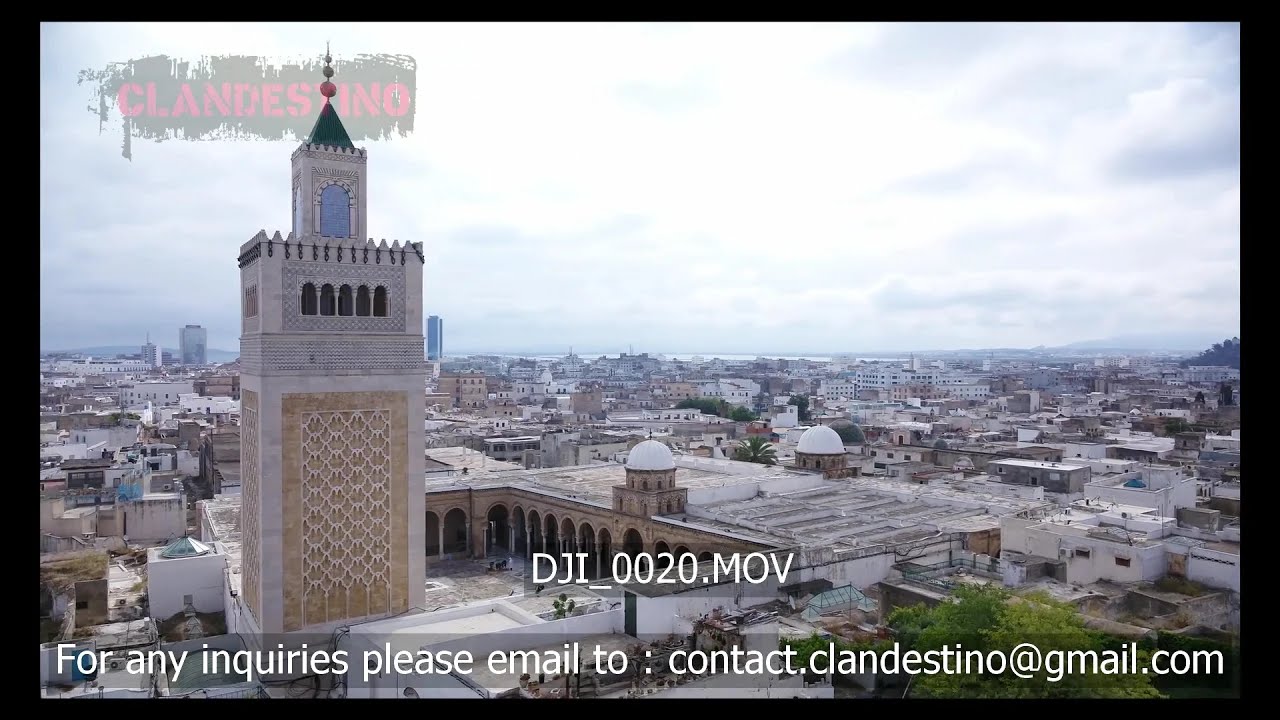The image portrays a bustling urban landscape under a gray, cloudy sky. Dominating the left side of the scene is a tall tower with a spire, possibly part of a church or mosque, adorned with ornate gold decorations and featuring blue, stained-glass windows. This tower stands in the center of a courtyard and is surrounded by a mix of low-rise buildings, warehouses, and a tree on the right front. In the distance, hills and a body of water are visible. Written in red capital letters in the upper left corner of the image is the word "Clandestino," or a similar variation. Additionally, text at the bottom of the image reads "DJI0020.MOV," followed by an email for inquiries: contact.clandiseno@gmail.com.